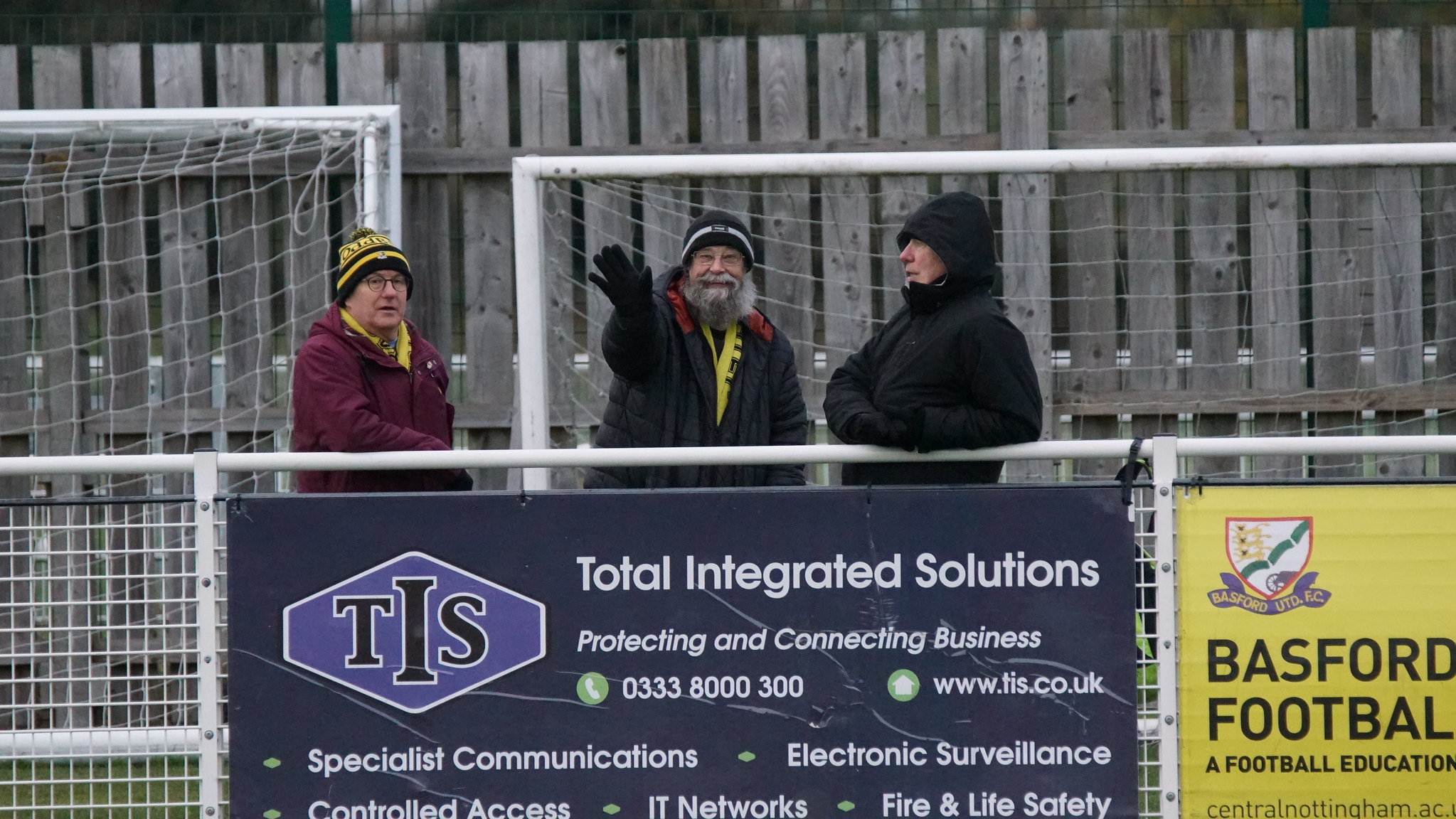The photograph is taken at the edge of a small outdoor soccer field, with three men standing behind a white fence. The man at the center, sporting a big grey beard, a beanie, gloves, and a heavy coat, is smiling and waving toward the camera with his right hand. To his right is a man dressed in a black coat with the hood up, leaning sideways on the white bar and looking off to the left. On the left side, a third man stands with a neutral expression, glasses, a black and yellow beanie, and a red coat, his arm also resting on the white bar. Behind them, several white-framed railings with netting and a tall wooden fence with vertical gray slats are visible, indicating the perimeter of the field. Directly in front of them, hanging on the white fence, are two signs: one on the left with a grey background and white lettering that reads "Total Integrated Solutions - Protecting and Connecting Business," detailing services such as specialist communications, electronic surveillance, controlled access, IT networks, and fire and life safety; the second sign on the right, in yellow, features the logo and name "Basford Football: A Football Education," with additional text "centralnottingham.ac" at the bottom.